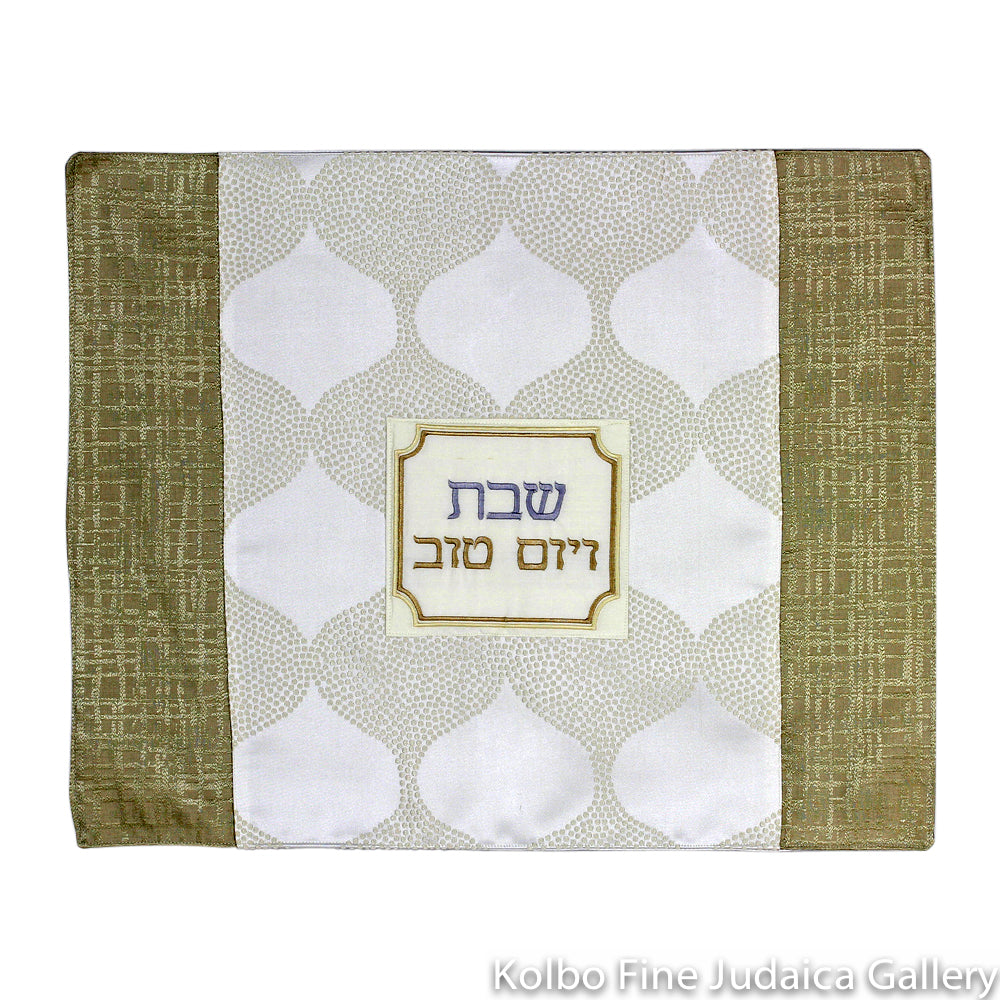This image features a sophisticated sales advertisement for a polyester Kahala cover designed for the Hebrew Bible. The cover displays a refined texture with a brown or light tan and gold checkered pattern on both sides. At the center lies a prominent white section adorned with dot-like globe designs exuding a futuristic vibe. Centrally positioned within this section is an off-white square with delicately rounded corners and a distinctive, bordered outline in brown, tan, and gold. This square houses intricate writing in a non-English script, showcasing an N, a backwards C, and a W in a vivid blue color. Below it, in gold, there's a sequence reading backwards C-7-0-space-0-7-apostrophe-7. At the very bottom of the image, the text "Kolbo Fine Judaica Gallery" is elegantly inscribed in grayish-white letters, emphasizing the artwork's cultural and artistic origins.